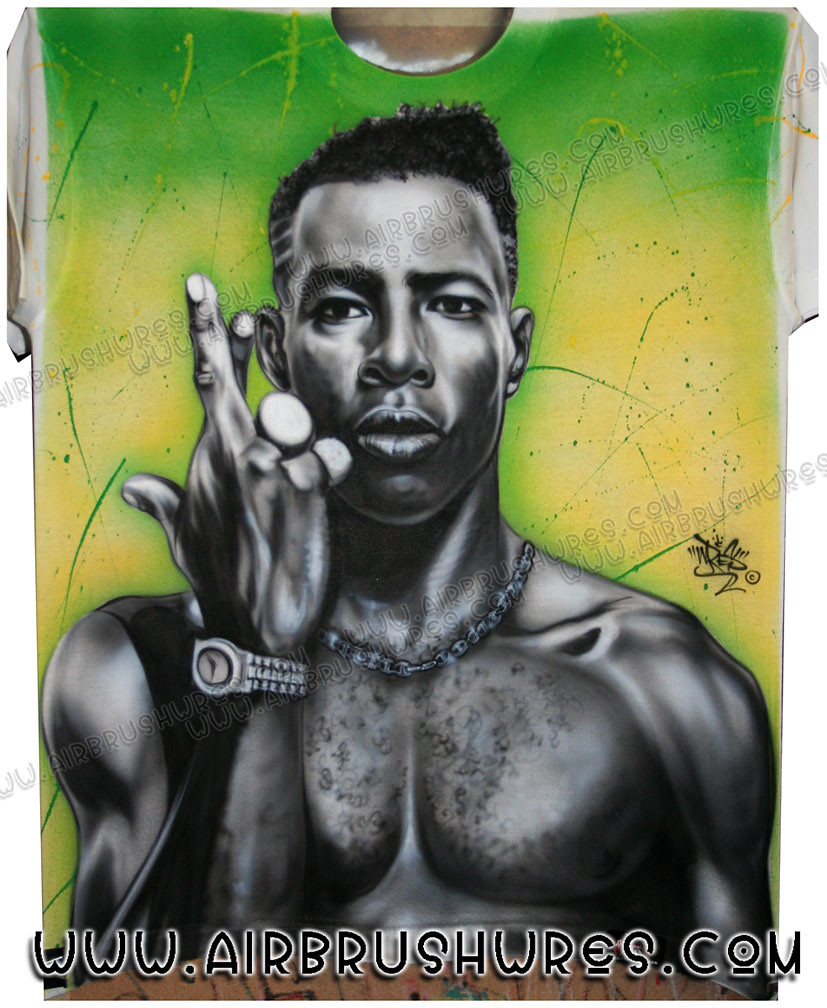The image showcases a vibrant piece of airbrushed artwork prominently displayed on a t-shirt. The primary focus is a detailed, airbrushed illustration of a shirtless man who is centrally positioned, taking up most of the image, leaving very little of the background visible. The background that is visible features a green gradient transitioning into yellow toward the bottom. The man in the artwork has a fade haircut with distinct stripes on the side of his head and is adorned with several accessories, including multiple rings on his fingers, a watch, and a chain necklace. He is depicted with his fingers crossed in front of him. At the bottom of the image, there is a web address, "www.airbrushrest.com," written in a stylized black font with white accents. The image appears to serve as an advertisement for an airbrush paint website, utilizing a dynamic palette of black, white, gray, green, yellow, and brown to create a striking visual effect.